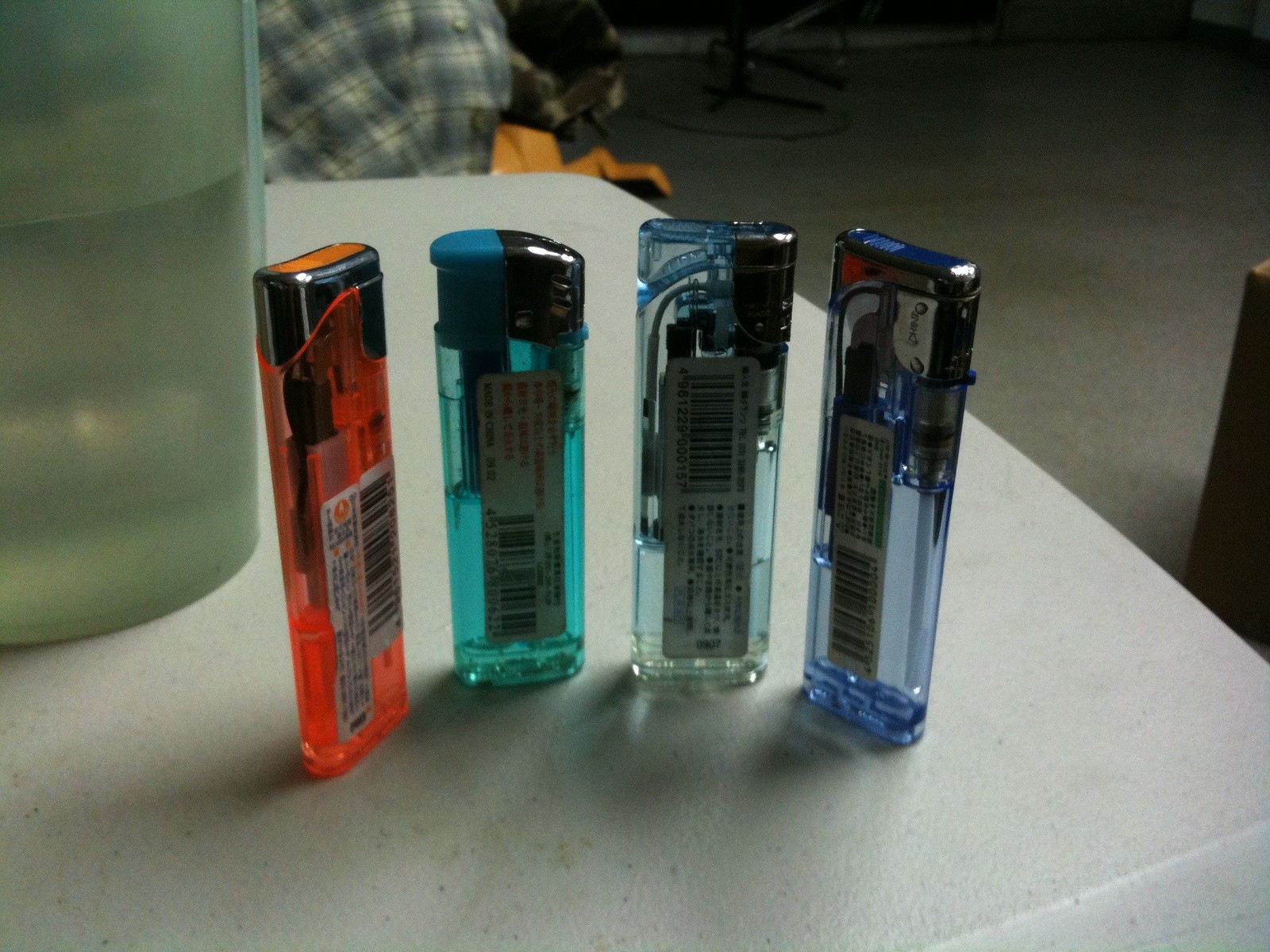This color image features a meticulously arranged composition on a white tabletop, reminiscent of those found in a lunchroom or cafe, set against a gray background. Dominating the center of the scene are four striking, tall plastic butane lighters, their somewhat transparent casings revealing the fluid levels inside. From left to right, the lighters showcase a spectrum of colors: an orange lighter with an orange button, a turquoise blue lighter with a blue button, a grayish-clear lighter with a black button, and a royal blue lighter with a matching blue button. Each lighter displays a white, long, and narrow label facing the camera, embellished with barcodes and text.

The lighters are positioned in a semicircle, casting long shadows toward the lower-left corner of the image. To the left side, slightly behind the lighters, stands a tall greenish-gray cylinder, possibly a jug or a glass, adding a touch of mystery to the scene. At the top left corner, the image captures a glimpse of a plaid or flannel shirt, suggesting the presence of someone seated at the far end of the table. This detailed arrangement creates a visually appealing and thoughtfully structured composition, highlighting each element's form and color.